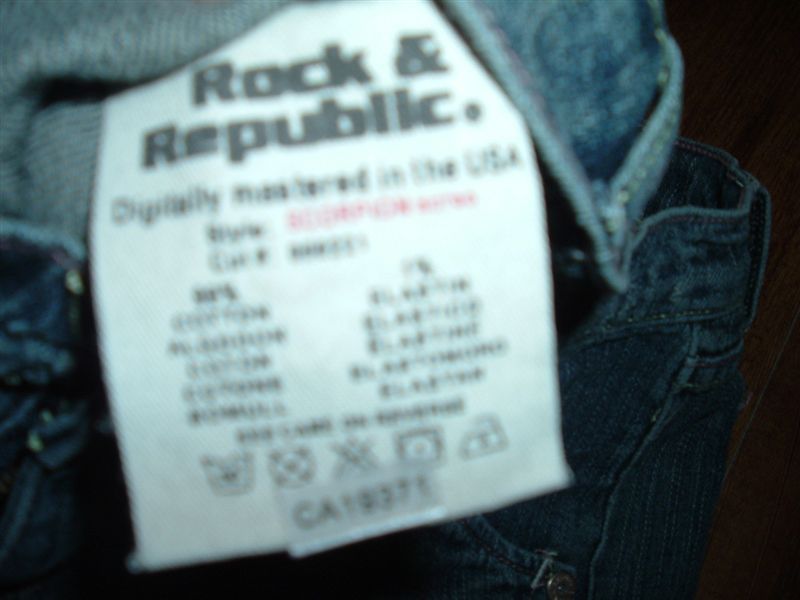A blurry image capturing a white care label, likely attached to a piece of clothing, set against a black and gray background. The top left corner of the frame features a light gray hue with a dark gray spot in its center. Surrounding the label, the left edge down to the bottom left corner and up the right side is predominantly black, with a small section of gray appearing to the right of the label. Despite the overall blurriness, "Rock and Republic" is discernible in black lettering on the label. The remaining text on the label is too blurry to be legible. At the bottom of the label, a row of five icons—typical for fabric care—indicates washing instructions, possibly for dry cleaning or other care specifics.